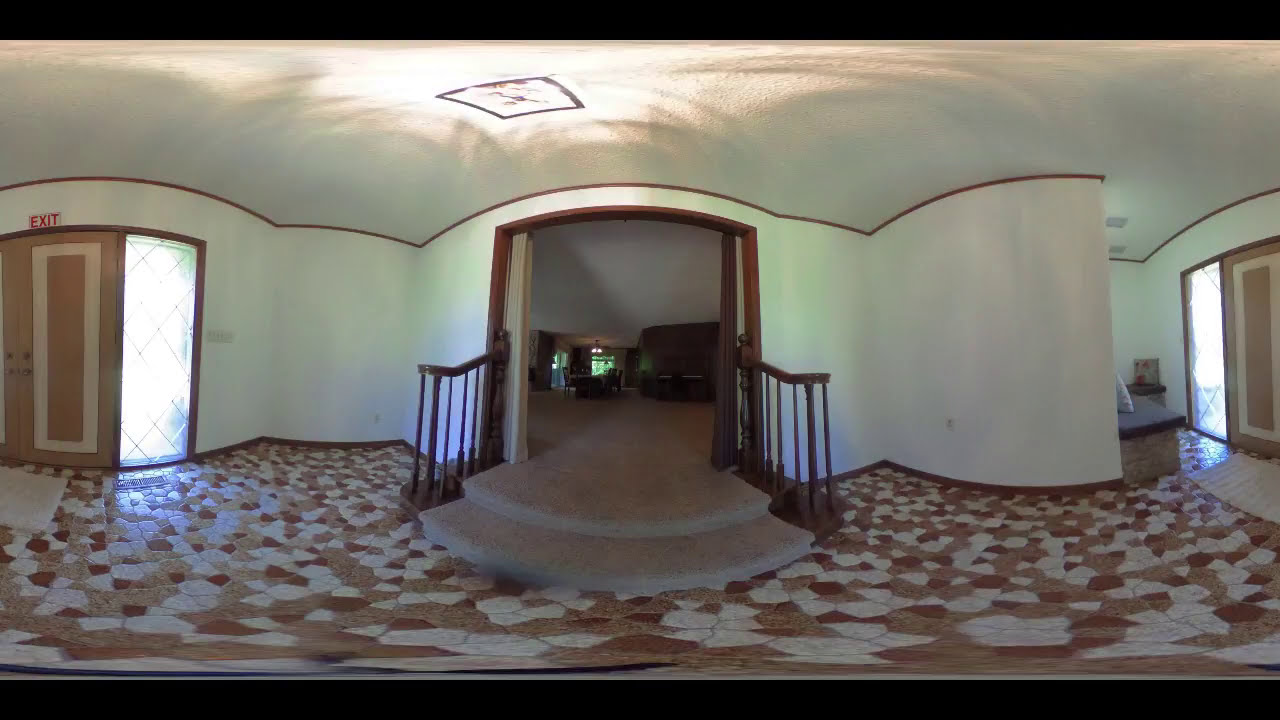This 360-degree photograph captures the interior of what appears to be a retro building from the 70s, 80s, or 90s, possibly a church, funeral home, or meeting hall. The image, distorted by the lens, showcases a tiled floor with a mosaic pattern of white, tan, and clay-red tiles. On the left side, an exit door with red lettering stands out, framed by glass panels. Centered in the image is a small, gray-carpeted staircase with dark brown wooden railings, leading into a larger, darker room in the background, illuminated by shadowy reflections on the curved ceiling. The room beyond is expansive and empty, with white walls adorned with thin brown trim. The ceiling remains white, contributing to the spacious and somewhat solemn atmosphere of the setting.